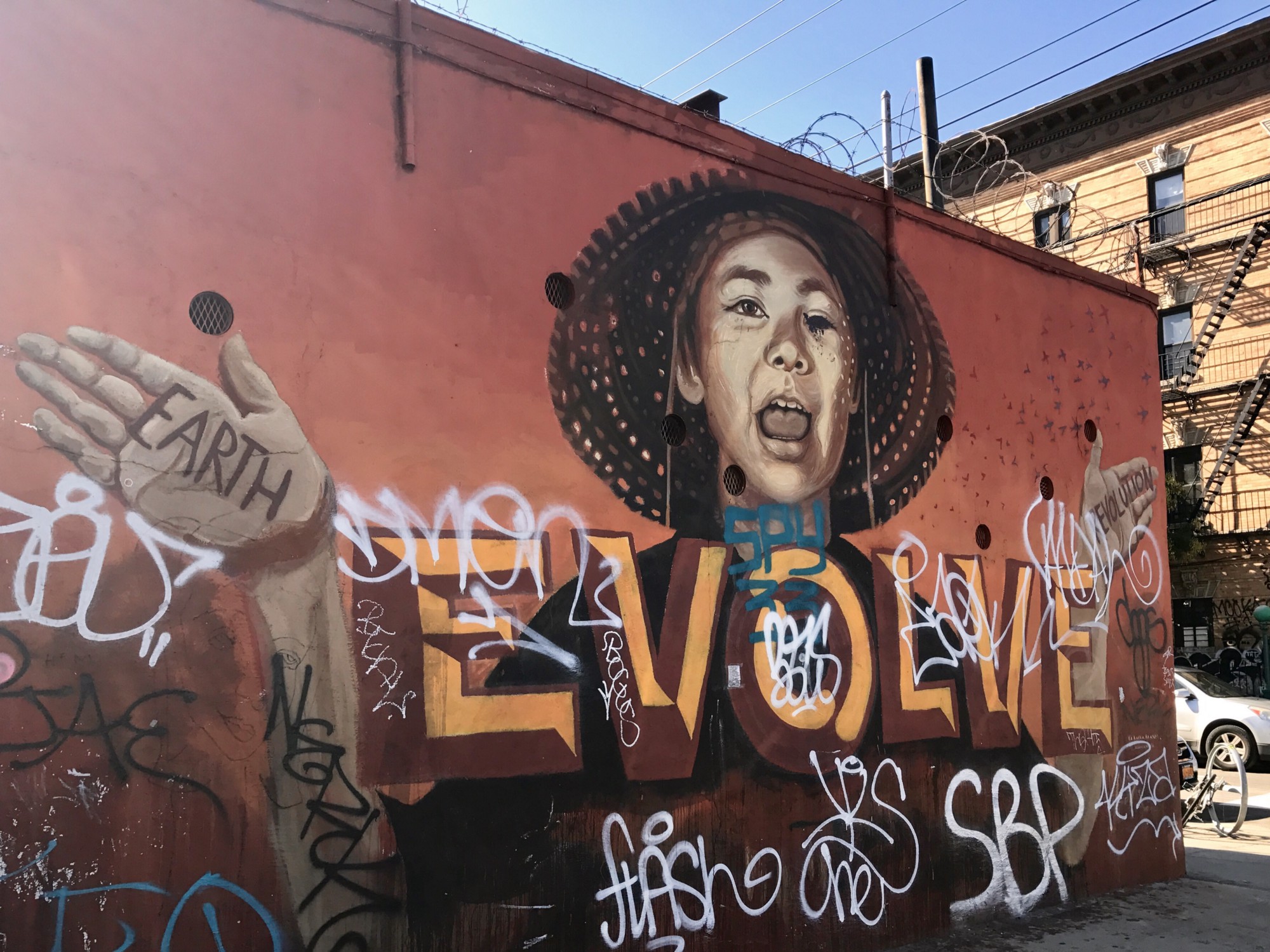The image depicts a vibrant urban mural spanning from the middle left to the middle right of the frame, set against a building backdrop. Dominating the mural is the image of a young teen with a tilted, sectioned hat featuring multiple lines of holes. The teen is posed with their arms outstretched to either side, hands flat with the left palm bearing the word "EARTH" and the right palm inscribed with "EVOLUTION". Beneath the figure, the words "EVOLVE" are prominently displayed in a blend of orange-yellow tones with a dark brown 3D effect. The mural's background is primarily red, layered with various illegible graffiti in white, black, and blue. Additional graffiti elements include the word "flash" around the left breast area and "SBP" near the right elbow. Surrounding the mural are elements of urban grit, including a barbed wire fence at the top of the building and a parked car near the building's base. The rich color palette incorporates sky blue, tannish beige, orange, brick red, white, yellowish beige, brown, gray, and darker blue, all contributing to the dynamic city scene.